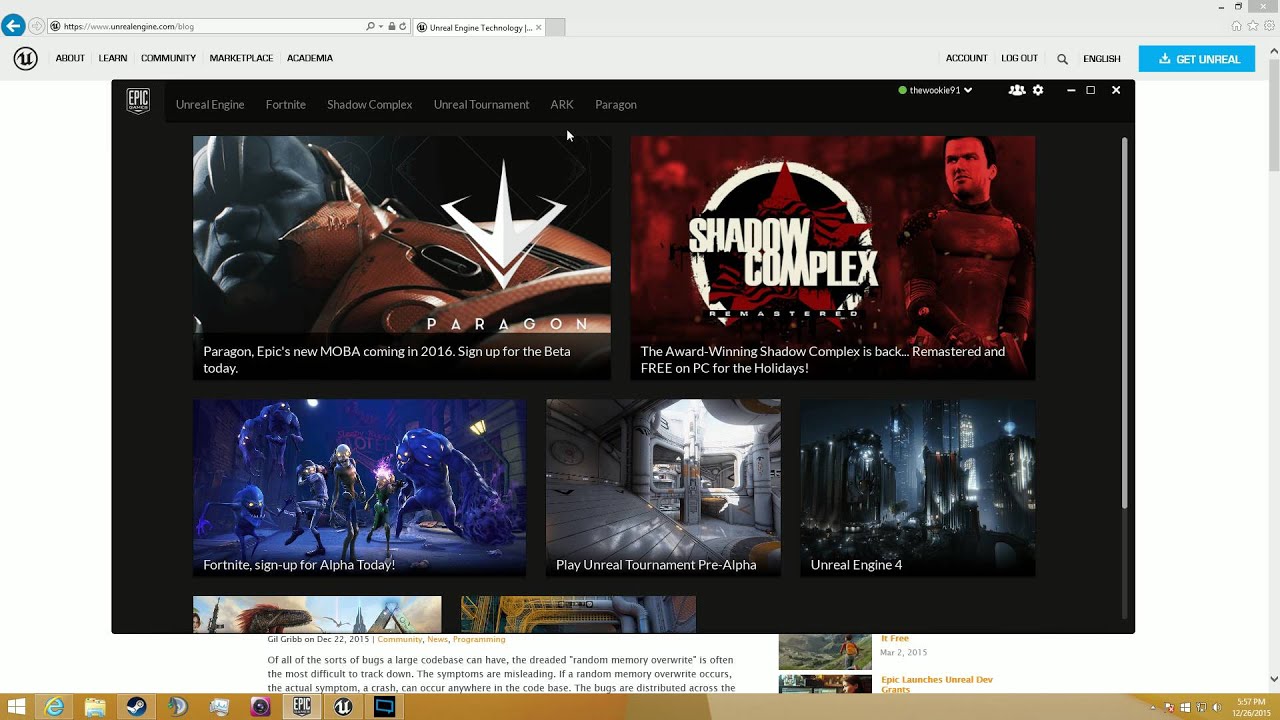This image showcases a sleek, dark-themed website for Epic Games, identifiable by a small Epic Games logo in the upper left corner. Dominating the top section is a black horizontal bar spanning the width of the page, featuring white text links for various sections such as "Unreal Engine," "Fortnite," and "Shadow Complex." Directly beneath this navigational bar are thumbnail images representing each game. Prominently, a large image depicts a character from "Paragon," showing a blue-skinned alien wearing a red space suit. Adjacent to it, a smaller icon for "Shadow Complex" features a man clad in Special Forces attire, gazing into the distance. Another thumbnail showcases vibrant characters from "Fortnite." These thumbnails serve as interactive gateways, allowing users to click and explore different games on the Epic Games website.